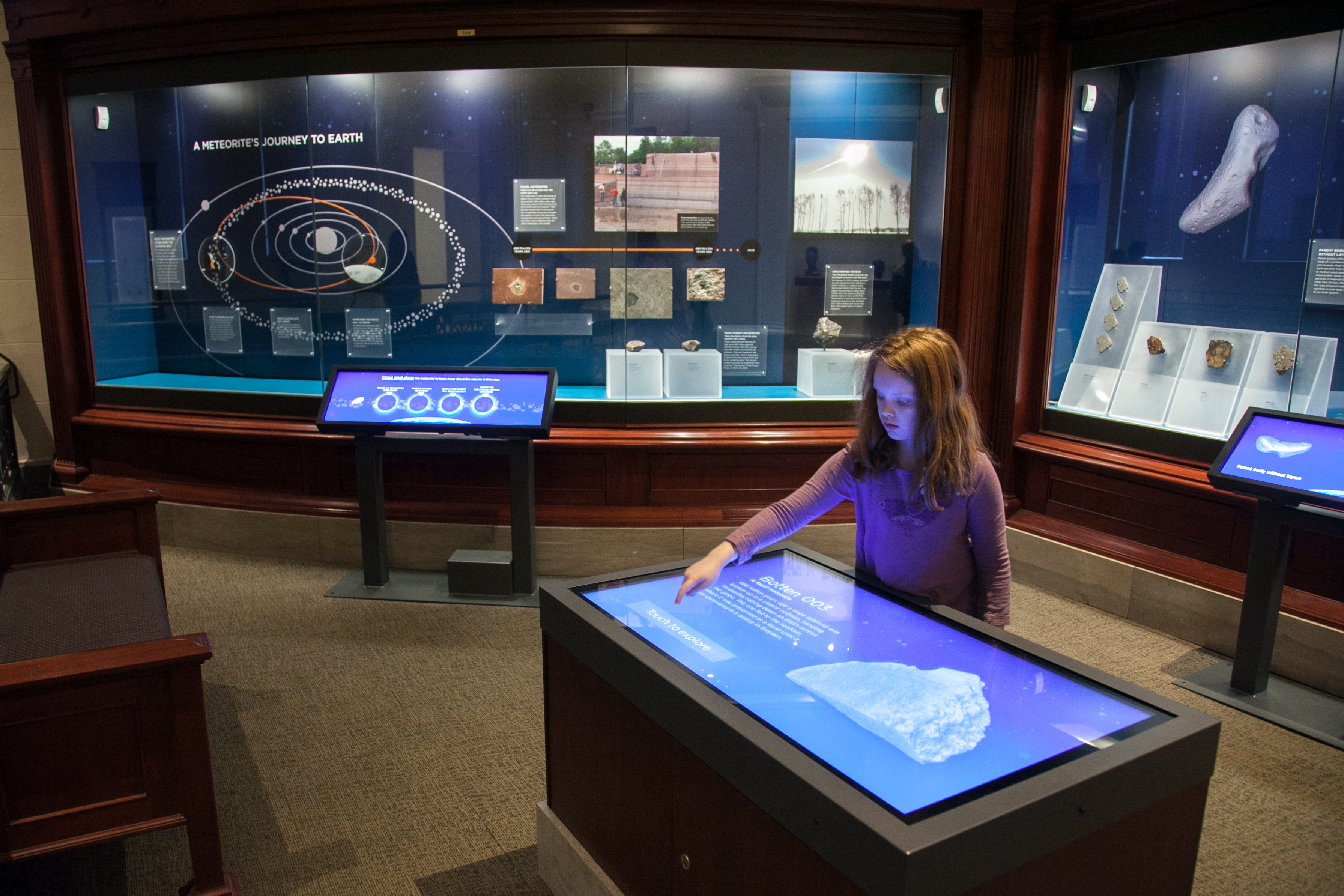The image showcases a young girl with long, brownish-red hair wearing a purple sweater, intently interacting with a touch screen on a wooden display stand in a museum. She has her right hand extended, pointing at a blue-lit display screen that features a white rock-like formation, likely a meteorite. The floor is carpeted, and there is a chair visible to the left side. In the background, glass-covered displays exhibit detailed graphics, including one illustrating a meteorite's journey to Earth with circular diagrams and scientific information about the solar system. On the right, there are more glass displays containing stones and meteorites, some presented on white box pedestals. The museum room is filled with additional stands and computer-like displays, contributing to the educational and scientific atmosphere of the setting. The scene is calm and unoccupied other than the focused girl, highlighting an environment dedicated to learning and exploration.